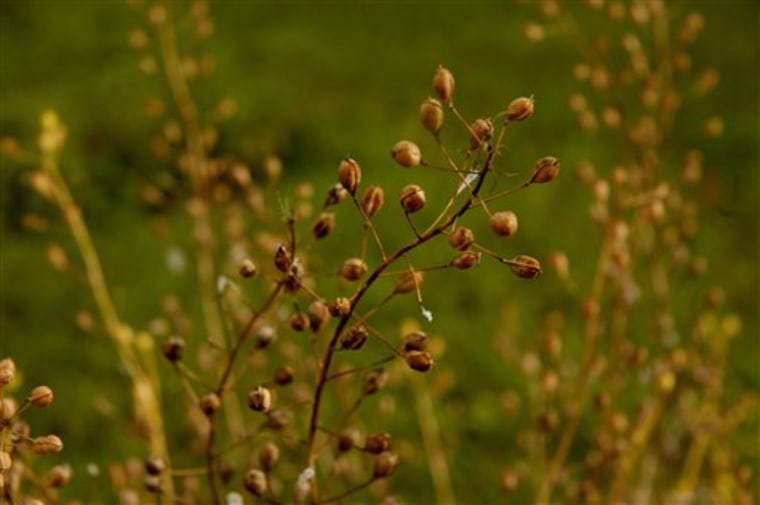This captivating close-up captures a vibrant outdoor scene in what appears to be a prairie, highlighting the intricate details of an autumnal plant with intriguing seed pods. The focal point of the image is a pair of slender, spindly stalks, each adorned with numerous small, rounded pods reminiscent of footballs or berries, displaying an array of warm, earthy tones—primarily shades of orange, brown, and hints of yellow. These pods, crisp and almost crunchy in appearance, stand in sharp focus against a backdrop beautifully softened by a bokeh effect. The blurred background is a lush blend of greens, suggesting surrounding grasses, enhancing the overall autumnal palette and creating a harmonious, natural setting.